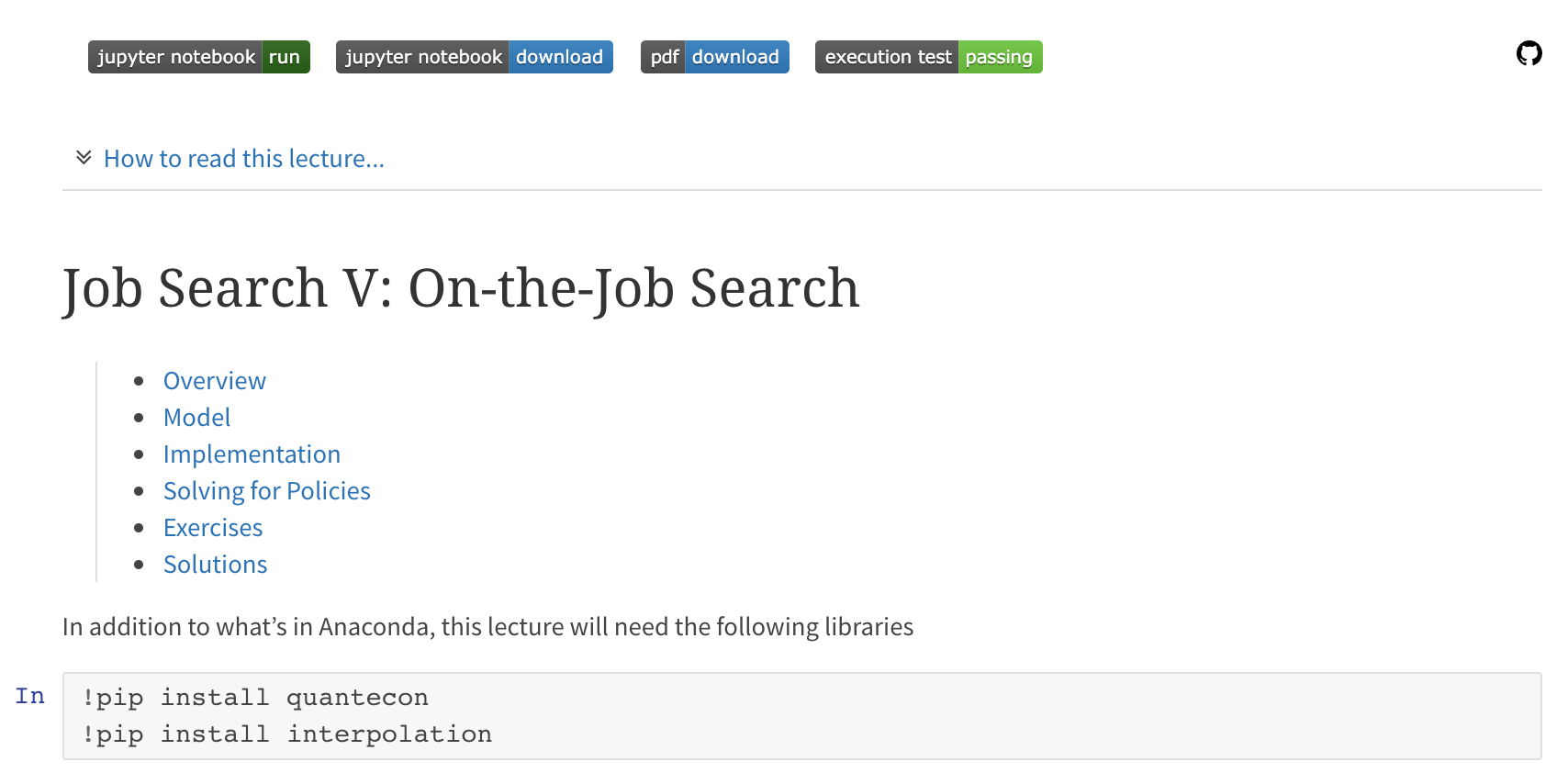In this screenshot of a GitHub repository, the GitHub logo featuring a white cat silhouette in a black circle background is prominently displayed. The repository, titled "Pageron Job Search," is dedicated to job search optimization and management. At the top of the page, various types of files such as Jupyter Notebooks, PDFs, and execution tests are listed, indicating diverse documentation and testing tools available within the repository. Below the main title "Job Search," there is a well-organized list of links presented in a bullet point format, including sections like Overview, Model, Implementation, Solving for Policies, Exercises, and Solutions. These links likely guide the user through different aspects of the project. At the bottom of the page, there are command line instructions provided for users to install the program on their local machines, facilitating easy setup and usage of the repository's resources.